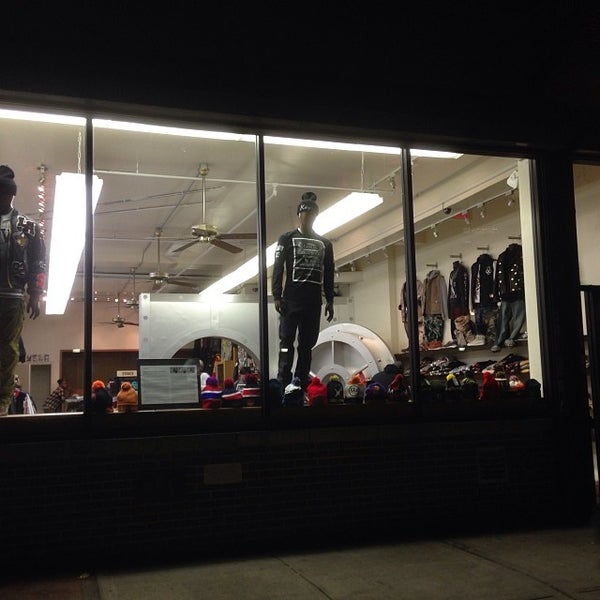The image captures the exterior of a shop at night. The scene is dimly lit, emphasizing the shop's tall glass windows embedded in a brick building, which exposes the brightly illuminated interior. Fluorescent lights, suspended from the ceiling, cast a stark glow over the space, accompanied by ceiling fans arranged in a row between the lights. Through the windows, an open door on the far wall reveals a group of people engaged in a meeting or discussion. A speaker stands at a podium while attendees sit attentively in chairs. 

A window display includes a mannequin dressed entirely in black attire, complete with a black beanie. Several more beanies are exhibited along the window's lower section. To the right, a variety of outfits, including shirts, jeans, and pullovers, are hung high against the wall, approximately 10-15 feet above the floor, adding a sense of verticality to the display.